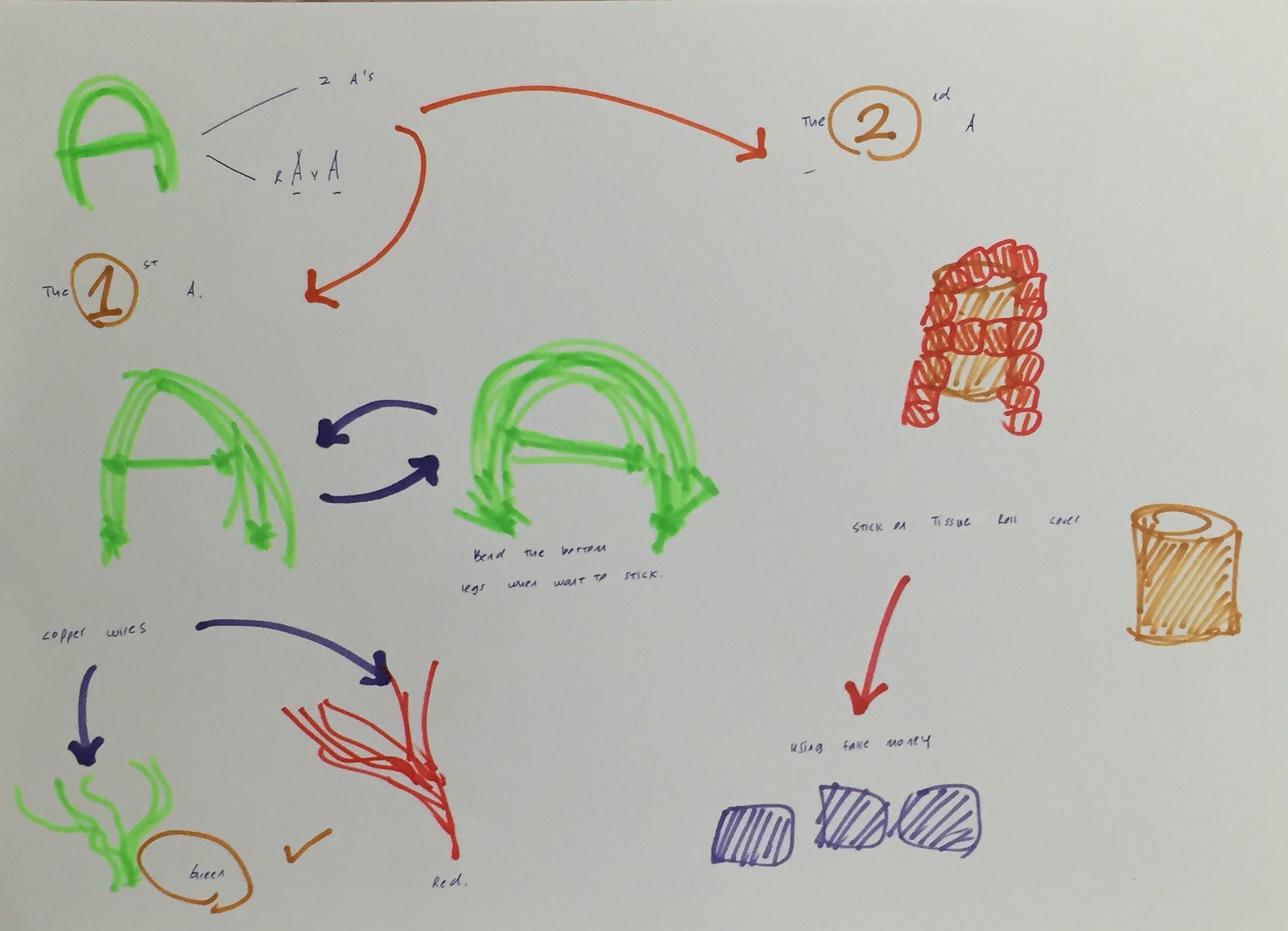This whimsical, childlike illustration, created with fine-point markers on a horizontally oriented, grayish sheet of paper, vividly captures an imaginative scene. In the upper left-hand corner, there is a unique, curvilinear symbol resembling an upside-down U with a line through it, which seems like an abstract representation of the letter A. Just below, a brown number 1 is encircled in a matching brown circle. Beneath this, another abstract "A" symbol appears with a right-pointing arrow beside it, directing attention to a green "A" next to it. This second green "A" has a blue arrow pointing back to the original "A," creating a looped connection between the symbols.

Below this section, wavy green lines, evocative of marine kelp or seaweed, add a touch of nature to the composition. Further down, another brown circle contains the word "beach," though it's possibly misspelled, accompanied by a brown checkmark. Adjacent to this, a segment labeled "red" features more plant-like designs, illustrated as red lines.

On the right side of the picture, the lower right-hand corner presents three irregularly shaped squares with lines through them, reminiscent of rocks. A red arrow descending towards these shapes emphasizes their presence, with the caption "Using Fake Money" written beneath the arrow, adding a quirky, narrative element to the artwork.